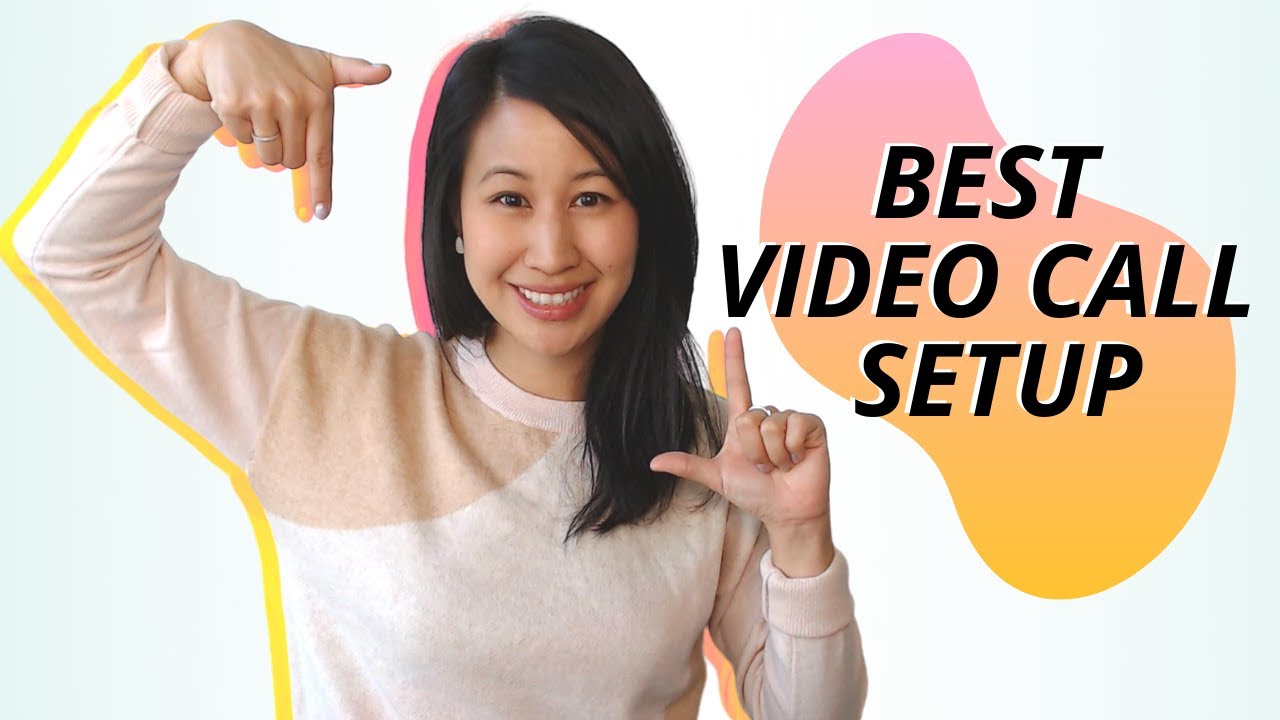In this visually striking advertisement photograph, a young Asian woman with long, straight black hair that drapes over her left shoulder is the focal point. She wears a stylish outfit featuring a white and light brown sweater, which is partially translucent over her right shoulder, creating an illusion similar to a strapless dress. The woman dynamically poses with her hands forming a picture frame; her right hand is raised with the index finger pointing down, and her left hand mirrors this with the finger pointing up, adding an engaging element to the composition. Encircling her left side is a vivid yellow outline, and the background behind her is dominated by a vibrant pink and tangerine gradient. To her left, in dark bold letters, the text "Best Video Call Setup" draws immediate attention. This combination of dynamic posing and bright, contrasting colors suggests the advertisement's intention to highlight a superior video call product or service, likely detailed in parts of the ad not visible in this image. The overall setting is minimalistic with a plain white background, accentuated further by the neon-like yellow and pink shadow that silhouettes her figure, contributing to the modern and eye-catching aesthetic of the graphic.